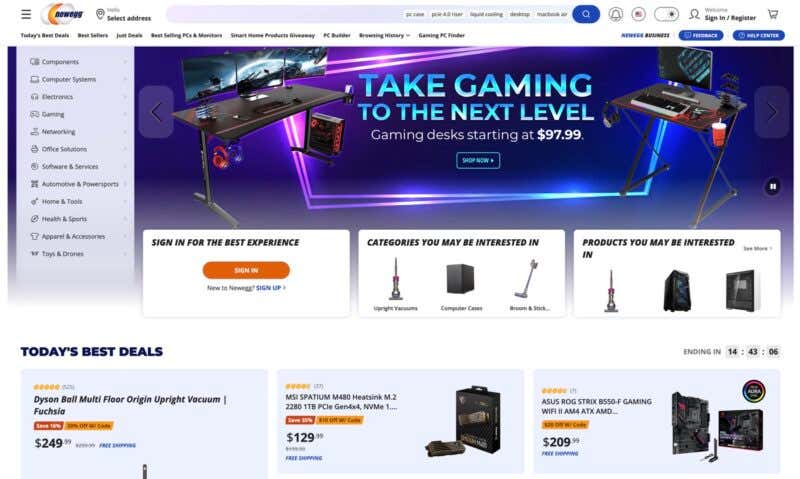This screenshot from the Newegg website's gaming section displays a detailed and visually engaging layout. The white header at the top features the Newegg logo in the upper left corner, with "Newegg" written in blue font beside three egg-shaped figures—two gray and one gold. 

Beneath the header, a menu bar displays several small-font items, including "Today's Best Deals," "Best Sellers," and "Best Selling PCs and Monitors," among others that are partially visible. 

Dominating the middle of the screenshot is a vibrant main graphic with a blue and purple gradient background. Metallic, iridescent text announces, "Take Gaming to the Next Level," while smaller white text below advertises "Gaming desks starting at $97.99." Flanking this central text are images of dark gray gaming desks.

Below the graphic, three rectangular boxes present additional options. The leftmost box invites users to "Sign in for the best experience," featuring a gold rectangle with rounded corners and a "Sign In" prompt in white. The middle box highlights "Categories you may be interested in," and the rightmost box suggests "Products you may be interested in."

Further down, another headline, "Today's Best Deals," precedes three showcased products. The left sidebar, set against a lavender background, lists various categories such as "Computer Systems," "Electronics," and "Gaming."